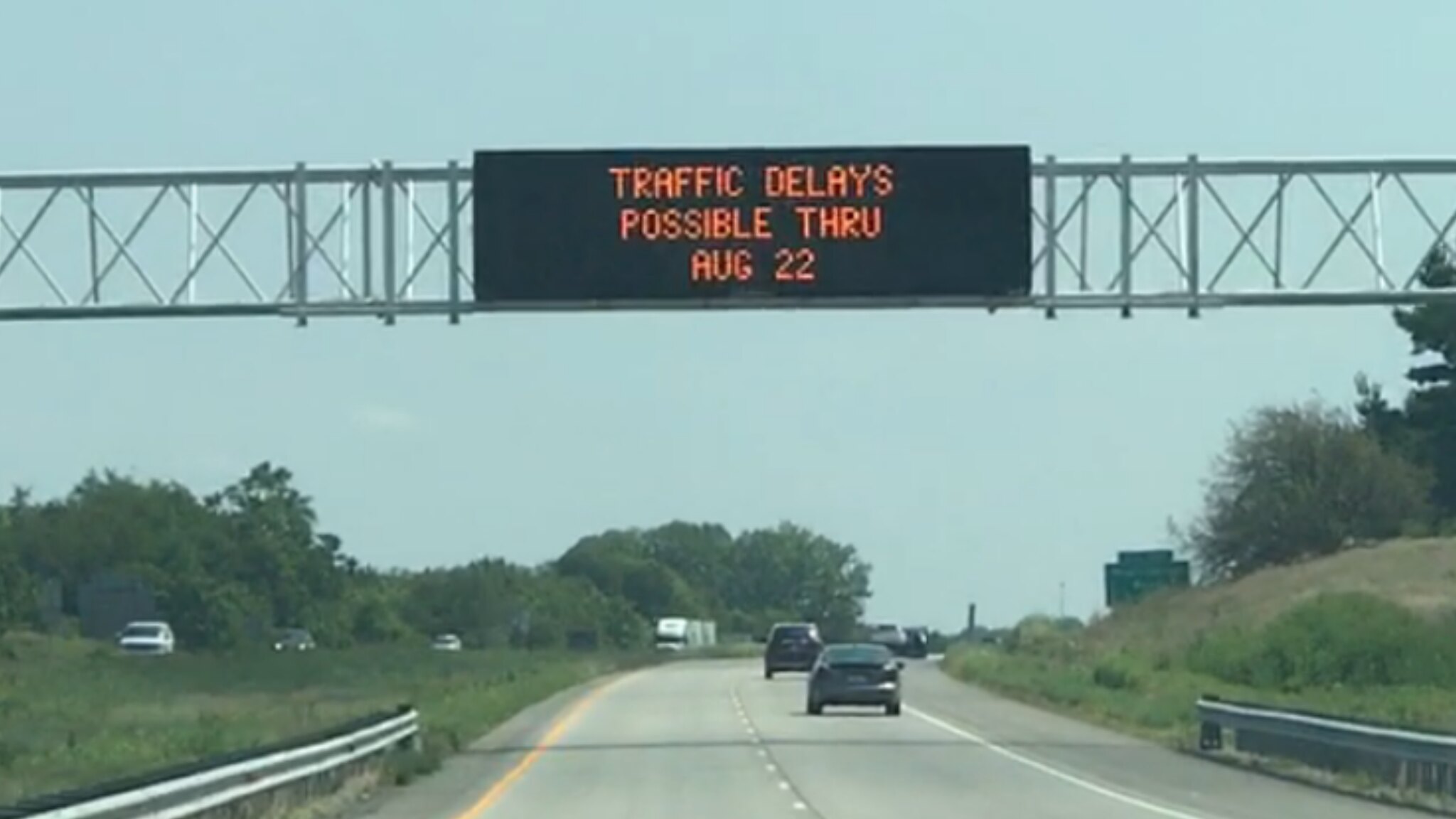The image depicts a busy highway with vehicles traveling in both directions. Prominently displayed at the top is an illuminated black sign with glowing red letters, warning of potential traffic delays through August 22nd. The highway itself is clearly marked with white dashed lines dividing the lanes and a continuous white line stretching along the center. A solid yellow line runs along the edge on one side of the road. Sturdy gray guard rails flank both sides of the highway, ensuring safety. In the distance, a large green highway sign is visible. The surrounding landscape is lush with green grass and an abundance of fully blossomed trees, creating a verdant and scenic backdrop.